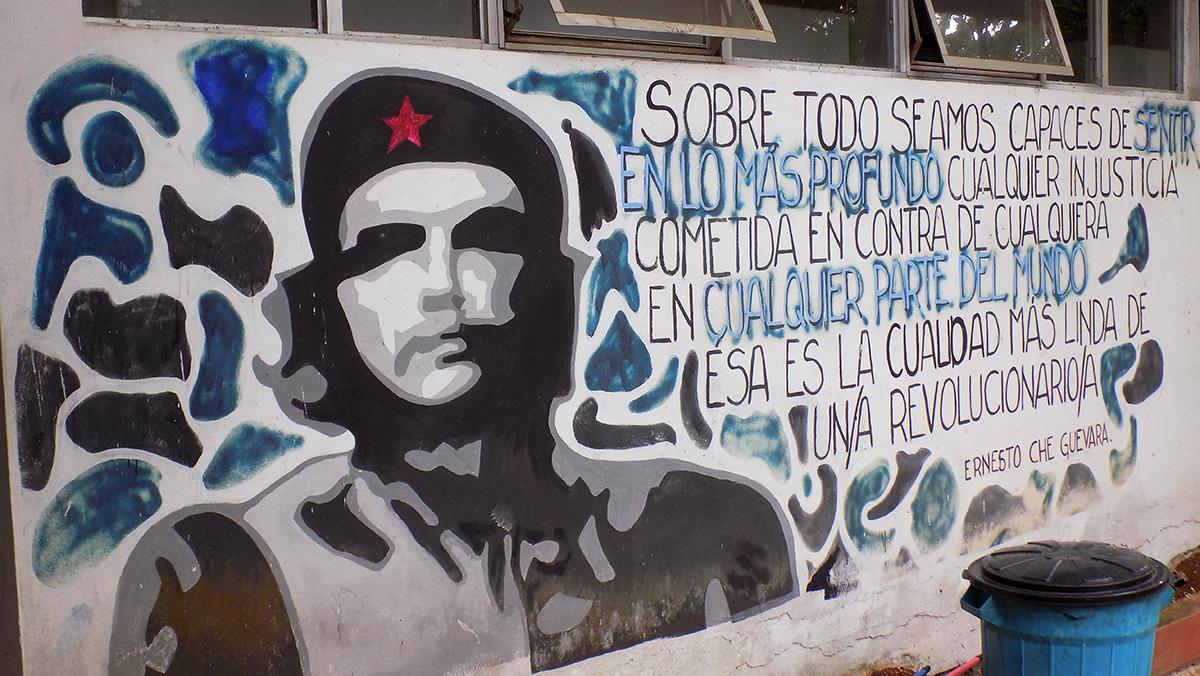The image showcases a large outdoor mural painted on a white wall, featuring the iconic revolutionary figure Che Guevara. His portrait, rendered in black, white, and various shades of gray, captures him from the shoulders up, dressed in what appears to be a military-style uniform. He is wearing his signature hat adorned with a red star. The mural includes an abstract background with shapes in blues, grays, and blacks surrounding his head and extending to the right. To the right of Che Guevara's portrait, there are six lines of text written in Spanish, though their content is not specified. At the bottom of the mural, his name, "Ernesto Che Guevara," is distinctly written. Below the mural, there are two crank-out windows, and a blue trash can with a black lid is positioned in front of the mural.